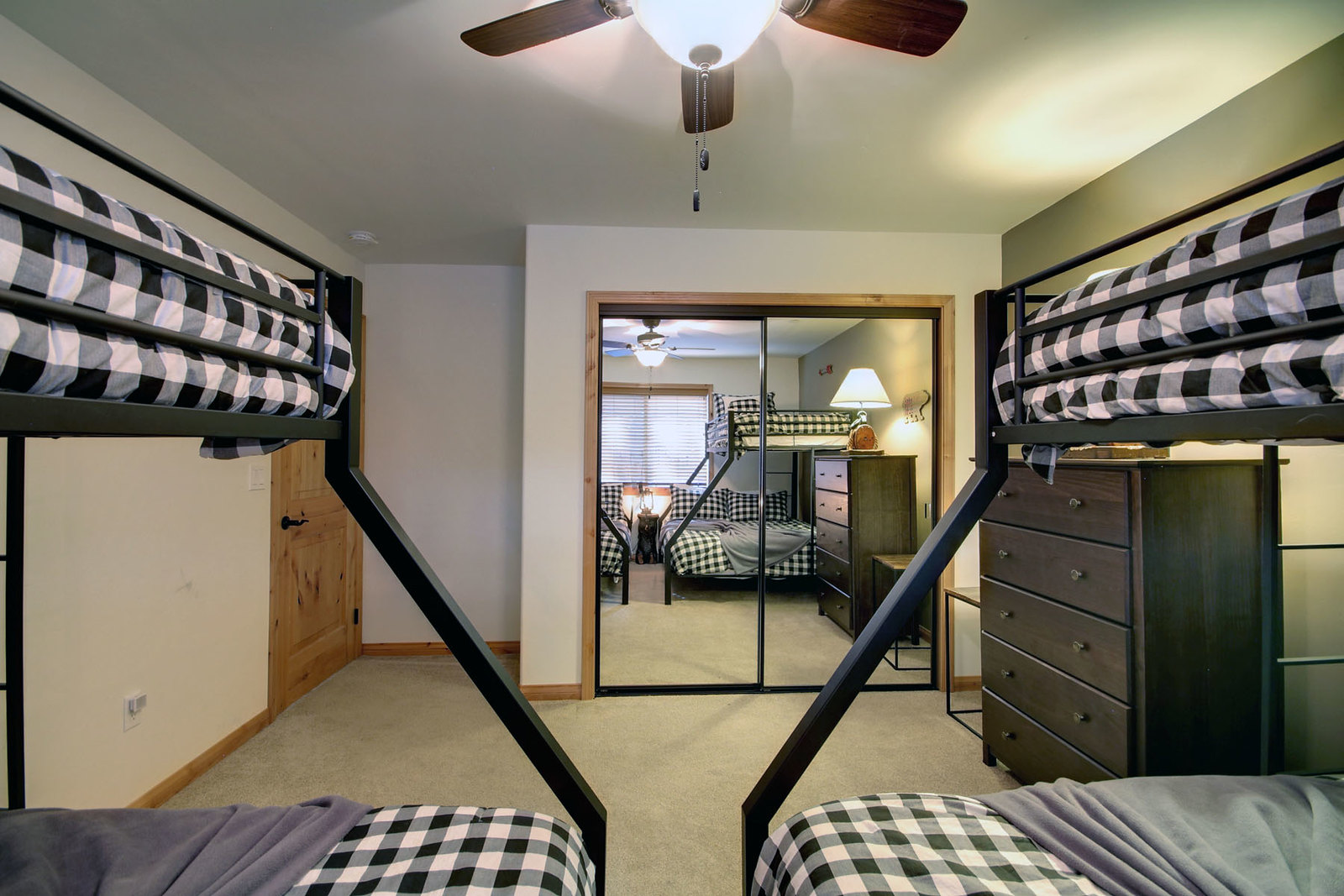This photograph captures a detailed view of a bedroom with two loft beds. Each bed frame is crafted from black metal and is accompanied by matching black and white checkerboard patterned comforters on both the top and bottom bunks, complemented by gray sheets underneath. The room features a beige carpeted floor, unpainted wood baseboards, and a barely green-tinged white wall. To the left, there's a closed door with a black handle. A wooden frame encloses a closed closet with sliding glass mirror doors that have black frames. Positioned between the closet and the bunk beds is a dark mahogany dresser with five drawers, atop which sits a lit lamp. The room is also illuminated by a ceiling fan with three visible dark wooden blades and dangling pull strings, one for the fan and the other for the light, which is switched on. Additionally, there is an alcove providing a subtle architectural detail.